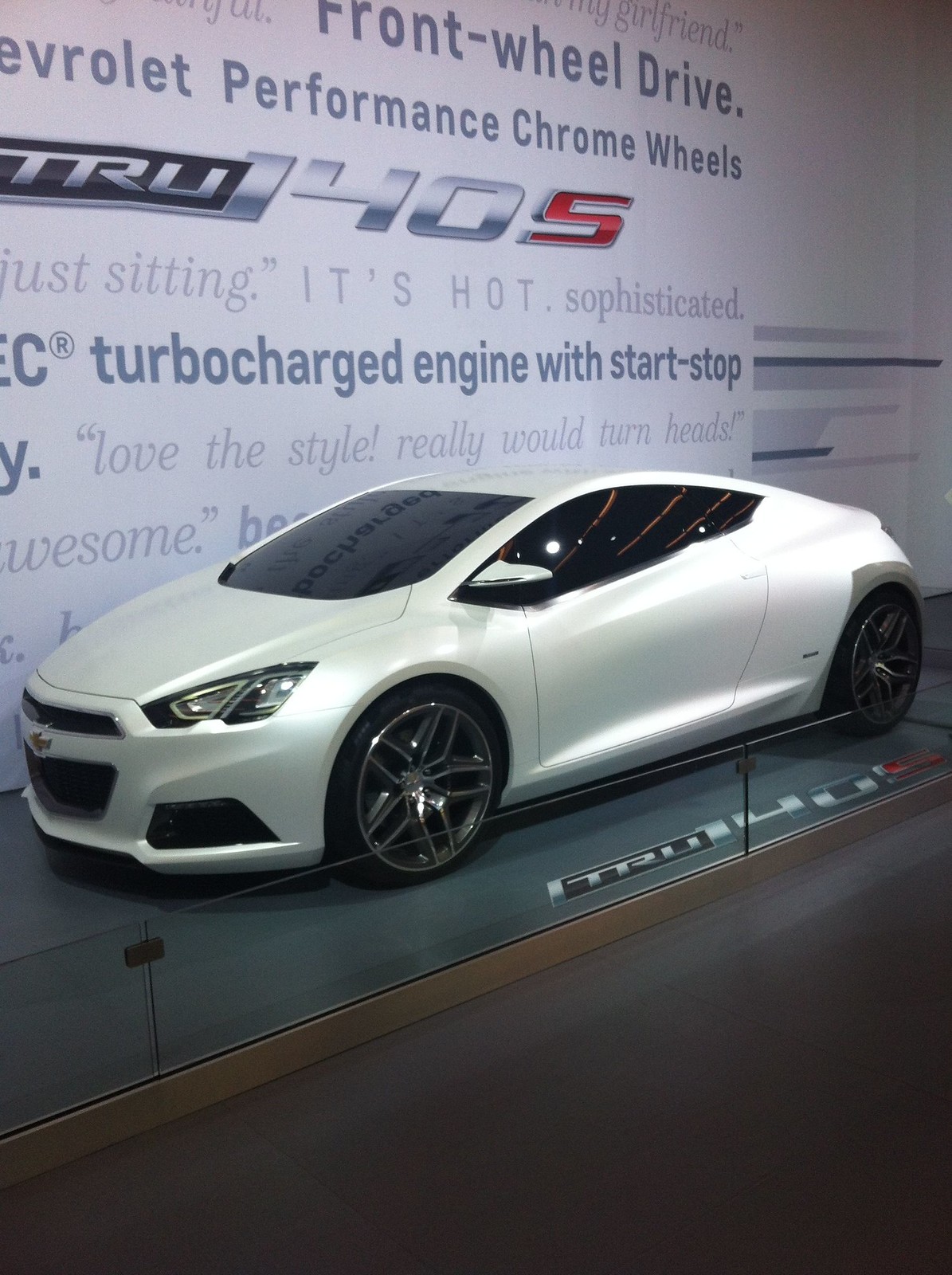The photograph, taken indoors at a well-lit event, showcases a sleek, silver Chevrolet sports car positioned behind a knee-high plexiglass display. The vehicle's pristine condition highlights its shiny, chrome wheels and black-tinted windows. Behind the car, a white backdrop adorned with promotional quotes emphasizes its features: "front-wheel drive," "performance chrome wheels," "turbocharged engine with start-stop," and "love the style, really would turn heads." Some of these quotes are even mirrored in the car's windshield. Notably, the model number "TRU1405" is prominently displayed on the floor beside the car, suggesting its designation. The image captures a side profile, with the hood visible to the left and the rear to the right, amid a bright and clear setting devoid of any people.